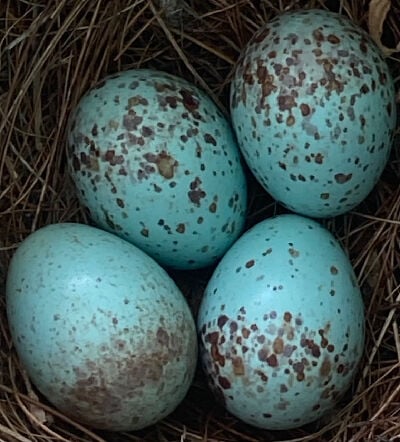This is a detailed photograph of a bird’s nest, featuring four blue eggs that are likely robin eggs, though their large size and distinctive speckling suggest they could be mistaken for something much larger, like ostrich eggs. The eggs exhibit a light robin egg blue color, each adorned with various amounts of brown, light brown, and gray speckles—giving them a speckled and slightly weathered appearance. The nest, constructed from an intricate mix of light and darker brown twigs, straw, and some dirt, provides a cozy backdrop. Positioned with two eggs at the bottom and two above, they show different speckle patterns, with the bottom left egg having a touch of brown at its base and the bottom right egg showcasing many more brown speckles. Overall, the image captures the serene beauty and intricate details of the nest and its precious contents.